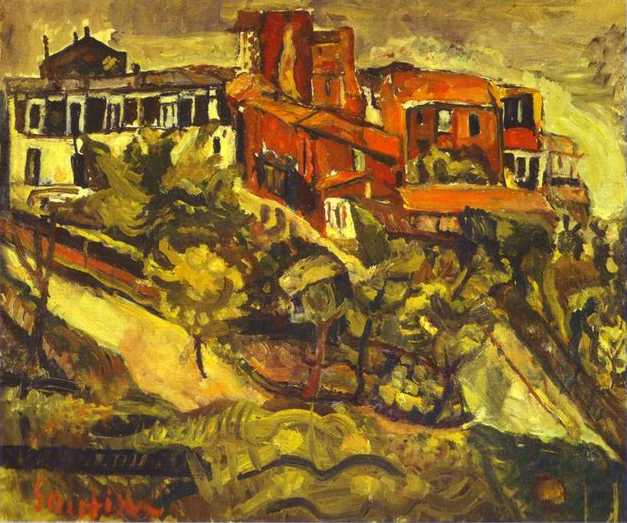This oil painting depicts a small village on a hillside, rendered in an abstract, stylistic manner reminiscent of Van Gogh. Dominated by subdued, goldish-orangish-yellow hues, the scene features a couple of lumpy, misshapen houses, adding to the painting’s whimsical and tilted aesthetic. On the left, there's an orange building with multiple levels and black windows, while a red-roofed, red-sided house stands prominently to the right. The foreground is filled with green trees, characterized by swirling, wavy lines and rooted firmly in the ground. Distinctive swirling black lines frame the various elements of the composition. The hillside stretches to the top of the painting, obscuring any view of the sky or sun. Although the painting is quite abstract and the details are hard to discern, there might be a signature in brighter red on the bottom left corner. Overall, the painting’s crude, imperfect lines and the vivid play of colors create an enchanting yet somewhat elusive depiction of a hillside village.